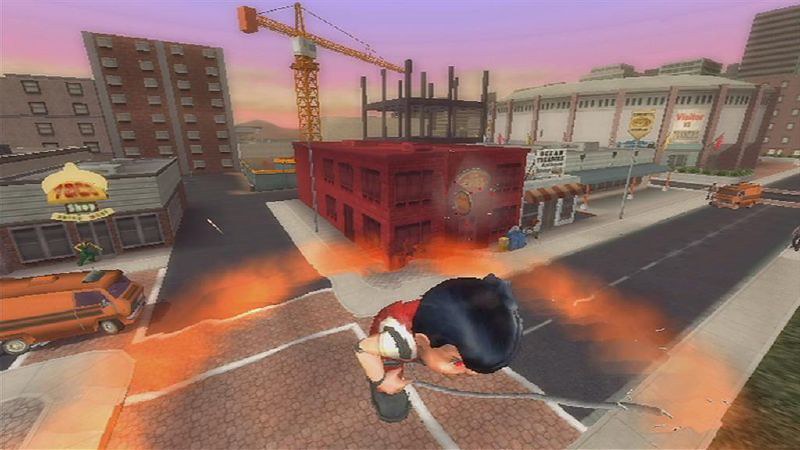This is a screenshot from a video game set on a bustling city street. Prominently featured in the center background is a large orange crane, indicative of ongoing construction. To the right of the crane stands the skeletal framework of a building under development, signifying the city’s continuous growth. Further back and to the top right, an arena can be seen, adorned with a white banner that has the word "Visitors" emblazoned in red.

Closer to the street on the right, there are two distinct buildings: a sizable red building and a smaller adjacent structure, adding to the urban landscape. A particularly striking element of the scene is a giant boy striding across a walkway, wielding a stick. He is dressed in a red outfit, and his black hair stands out against the colorful backdrop. On the left side of the road, an orange van is patiently waiting at a stop sign, contributing to the dynamic yet paused moment captured in the game.